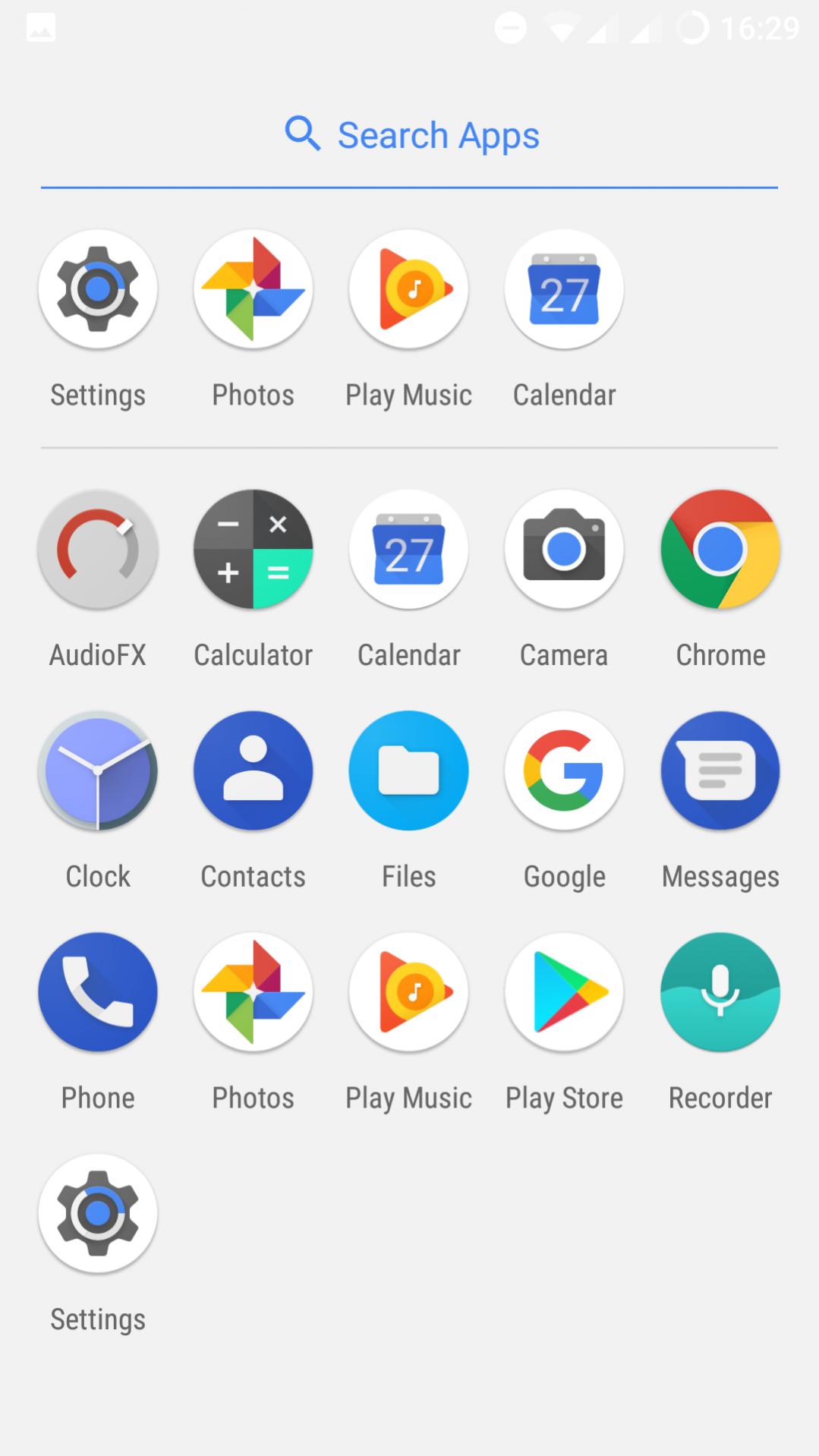This is a detailed screenshot of the main home screen of an Android phone. At the top right of the screen, white text displays the time "16:29." To the left of the time, there is a loading circle icon, followed by a Wi-Fi signal icon. On the top left, various system icons are also present.

Central to the image, "Search Apps" is prominently displayed in blue text with a matching blue magnifying glass icon to its left. Below this, a thin horizontal blue line marks a division.

Directly underneath, there are four primary app icons arranged from left to right: Settings (represented by a gear symbol), Photos (depicted with origami-like shapes in yellow, red, green, and blue), Play Music (highlighted by a triangular play button), and Calendar (featuring a classic calendar image).

Further down, a grid of app icons is organized in rows:

1. **First row from left to right:** 
   - AudioFX
   - Calculator
   - Calendar
   - Camera
   - Chrome

2. **Second row from left to right:** 
   - Clock
   - Contacts
   - Files
   - Google
   - Messages

3. **Third row from left to right:** 
   - Phone
   - Photos
   - Play Music
   - Play Store
   - Recorder

4. **Fourth row from left to right:** 
   - Settings

Overall, the screenshot provides a comprehensive view of the primary and secondary apps available on the Android phone's home screen.